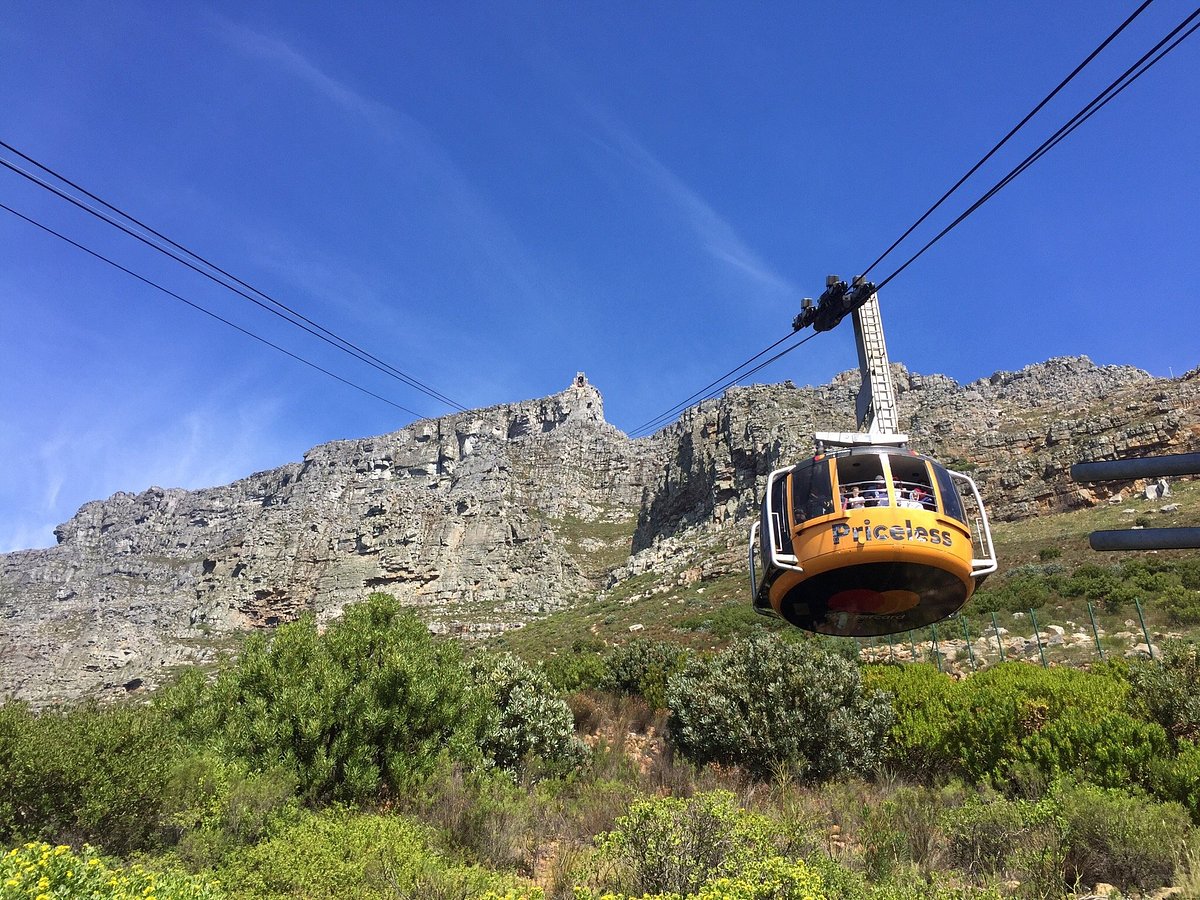The image captures a striking scene of a yellow and white gondola labeled with the word "PRICELESS" in black and a MasterCard logo at the bottom. The gondola, containing multiple people who are looking over its railing, is seen from a low-angle perspective, suspended from one of two cable lines against the backdrop of a mountainous landscape. The rocky terrain dominates the middle half of the image, while the top half features a clear, blue sky with minimal clouds. Below the gondola, the field is a mix of grass, trees, and brownish, semi-desert terrain, adding a contrasting earthy element to the scene.